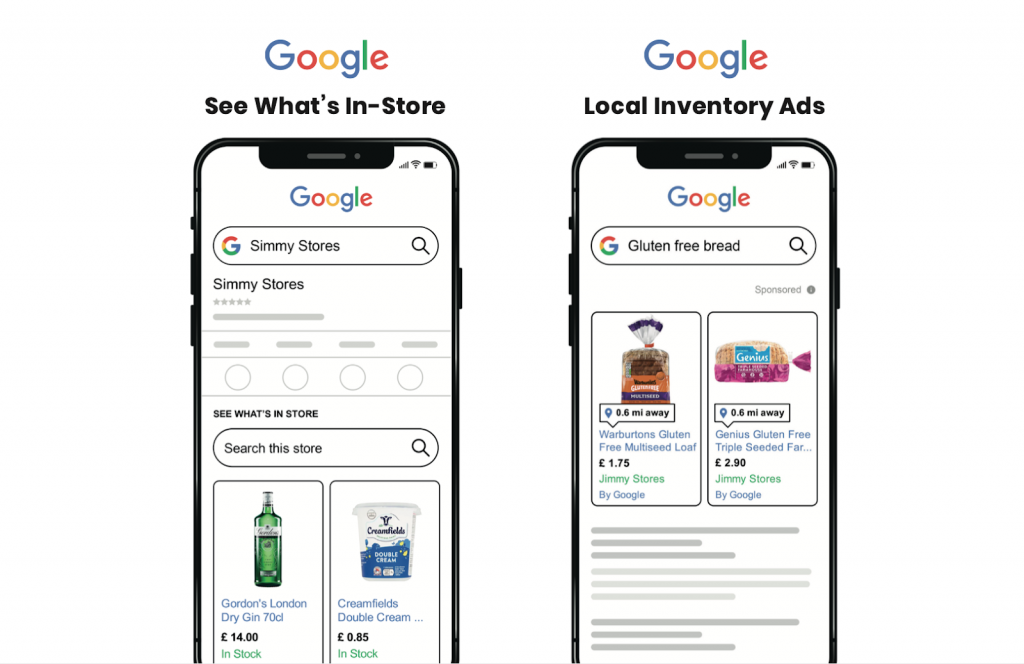**Caption:**

A comparative screenshot of two mobile phones displaying different Google search results for local inventory ads. 

- **Left Side:** 
  - **Header:** "Google - See What's In Store"
  - **Search Query:** "Simi stores"
  - **Results:**
    - **Item 1:** Gordon's London Dry Gin priced at £14, available in stock with an accompanying image.
    - **Item 2:** Creamfields Double Cream priced at £0.85, shown as in stock with an accompanying image.

- **Right Side:**
  - **Header:** "Local Inventory Ads"
  - **Search Query:** (Blurred, but showing local inventory results)
  - **Results:**
    - **Item 1:** Warburton's Gluten-free Multi-seed Loaf located 0.6 miles away, priced at £1.75, with an image.
    - **Item 2:** Genius Gluten-free Triple Seeded Bread, also 0.6 miles away, priced at £2.90, with an image.

Both phones showcase different layouts and functionalities of Google's local inventory ads, helping users find store-specific items with availability and pricing details. The rest of the content on the right side is blurred out.